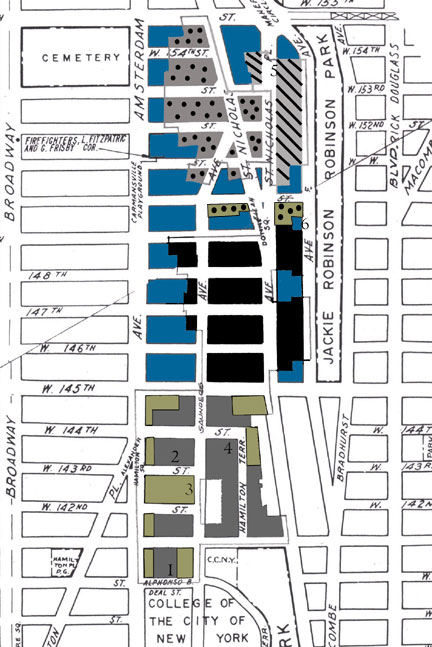This image is a detailed scan or high-quality photo of an old map, specifically of the College of the City of New York, likely situated in upper New York City near Harlem. The map predominantly showcases the city's grid layout with a focus on streets and buildings, featuring familiar names like Broadway, Amsterdam Avenue, and West 145th Street. The architectural outlines are primarily rendered in black and white, while certain regions are highlighted in blue and brown, possibly indicating areas of significance. Notable landmarks, such as Jackie Robinson Park and a cemetery located in the upper left corner, are clearly labeled. Additionally, the map contains specific annotations like 'Firefighters L Fitz Zipric and G Fritz B Corps,' connected by lines, hinting at historical or functional elements. Though the map's primary intention appears to be illustrating streets and significant structures, the exact purpose of the colored zones remains unspecified.